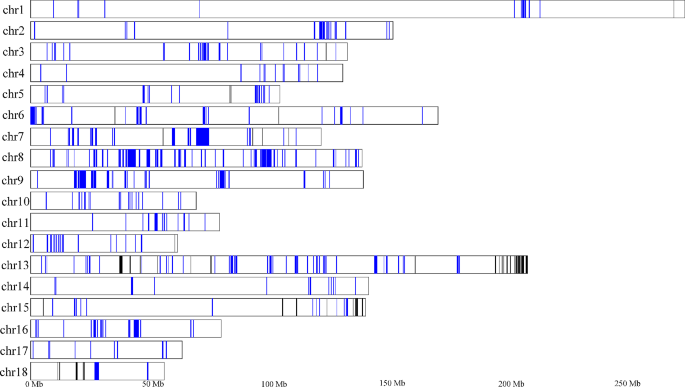This image features a detailed scientific diagram likely associated with genetic sequencing or chromosome mapping. The vertical axis on the left side is labeled with CHR1 through CHR18, which possibly stands for chromosomes 1 through 18. Across each row, which represents an individual chromosome, are long white strips interspersed with randomly spaced blue markings. The horizontal axis at the bottom is a scale ranging from 0 to 250 MB, though the exact unit seems ambiguous; it could denote a genetic measurement unit rather than computer megabytes. The layout suggests a comparison or sequencing chart where CHR1 extends beyond the 250 MB mark, and CHR 18 is the shortest, around 50 MB. Each chromosome strip varies in the number and arrangement of blue markings, hinting at diverse sequencing data or genetic markers.